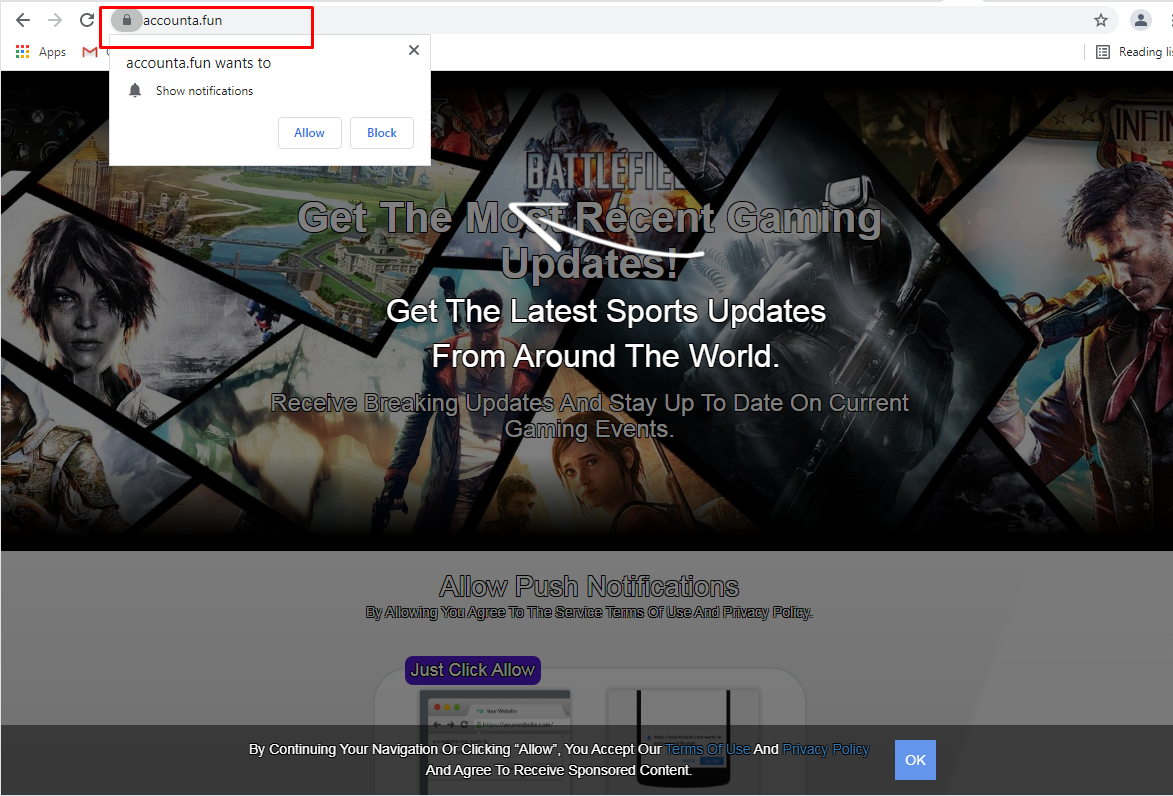The image depicts a computer screen, showcasing a web browser. In the top left corner, there are navigation icons: a left-facing arrow for going back, a right-facing arrow for going forward, and a circular arrow for refreshing the page. A red outline highlights the browser's search bar, which contains the URL "accounta.fun," accompanied by a small lock icon, indicating a secure site.

Below this red-outlined search bar, a notification prompt is visible, asking if the user wants to receive notifications from "accounta.fun." The prompt features a bell icon and offers two options: "Allow" or "Block."

Further down the screen, there is an advertisement for a game titled "Battlefield," highlighting options to "Get the most recent gaming updates" and "Get the latest sports updates from around the world." An arrow points to some feature on the left, where the image of a futuristic, space-age girl with robotic elements is displayed, suggesting a theme related to video gaming and advanced technology.

Below this image, there is a statement informing users that by allowing push notifications, they agree to the service's terms of use and privacy policy. Toward the bottom of the prompt, a small button with the word "OK" is visible, concluding the notification prompt.